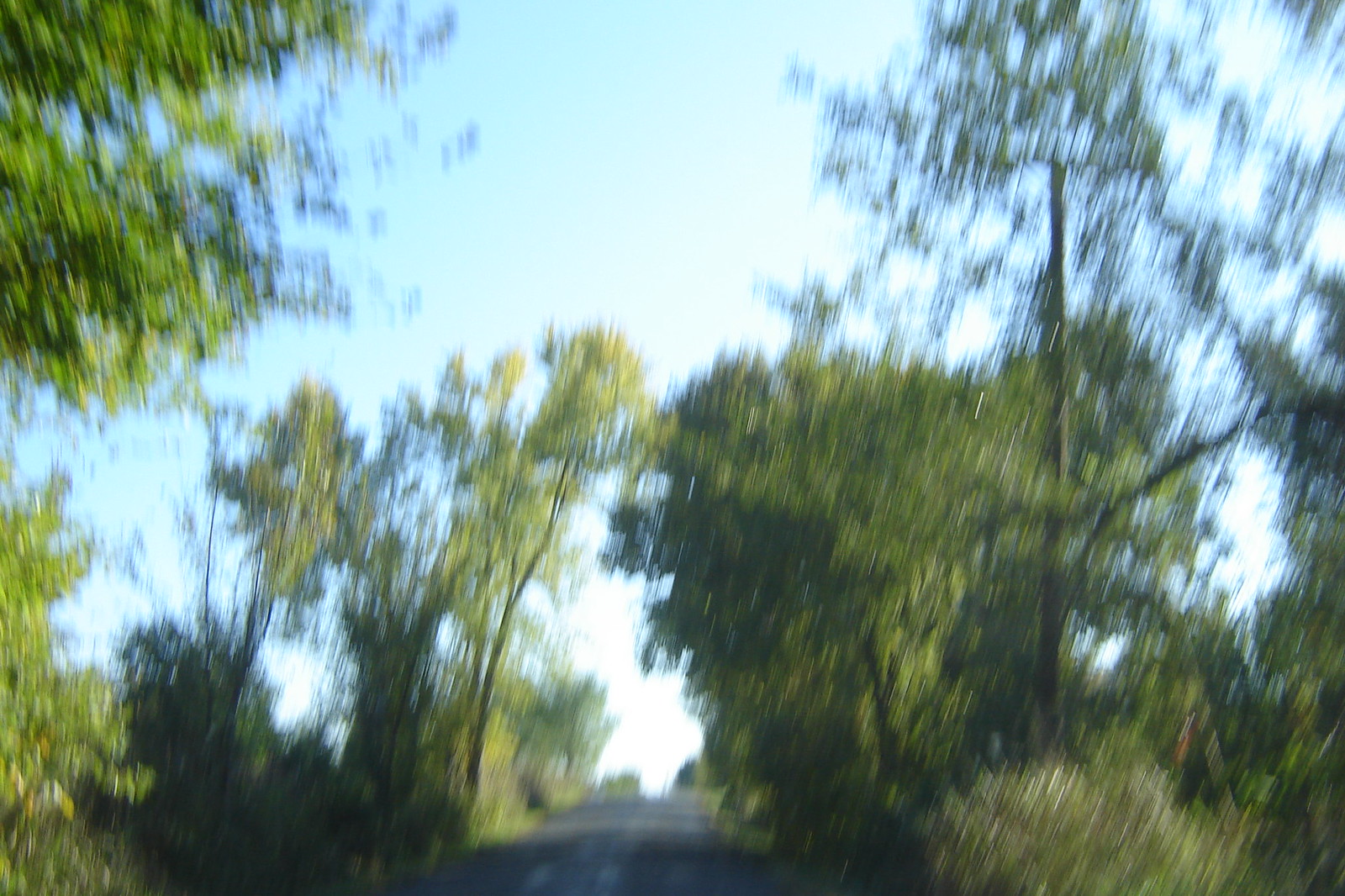The image captures an outdoor scene, albeit blurred and grainy, taken during daylight hours. The sky, a mix of white and blue hues, forms the backdrop of the scene. A line of leafy trees extends from the upper left corner, dips towards the bottom, and continues to the upper right. These trees display a variety of green shades, from deep hunter green to vibrant lime green. In the center of the image, a gray, paved road cuts through the landscape, shaded by the overhanging trees and disappearing into the horizon. On the upper right, a solitary pine tree stands out, surrounded by what appear to be oak trees. This pine tree is bare in its lower three-quarters, with its needles concentrated towards the top, creating a stark contrast against the sky peeking through its branches.